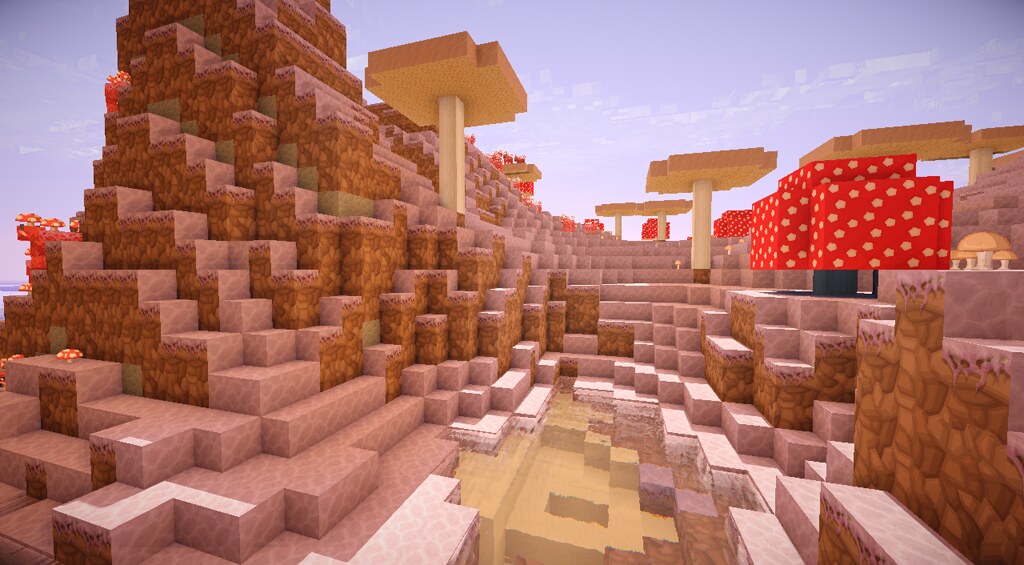This is a detailed screenshot taken from the video game Minecraft, easily identifiable by its characteristic world composed entirely of cubes, squares, and rectangle shapes. The image depicts a mushroom biome, a unique and vibrant landscape known for its distinctive vegetation. Several large mushroom trees populate the area; the brown mushrooms stand tall with light brown stems, while the shorter, squat red mushrooms feature dark blue stems and white spots.

The terrain itself mirrors this mushroom-themed palette, with a mix of darker and lighter brown hues. Scattered across the landscape are smaller mushrooms, much less imposing than their large counterparts, likely the type that players would quickly harvest. A small body of water, either clear or slightly tinged brown, is also visible.

The sky, a clear blue with some clouds, suggests either sunrise or sunset, or perhaps it's about noon. On the left-hand side, there are red cows, commonly known in the game as "Mooshrooms," with mushrooms growing on their backs. The scene is one of fantasy and natural beauty, capturing the unique essence of Minecraft's mushroom biome.